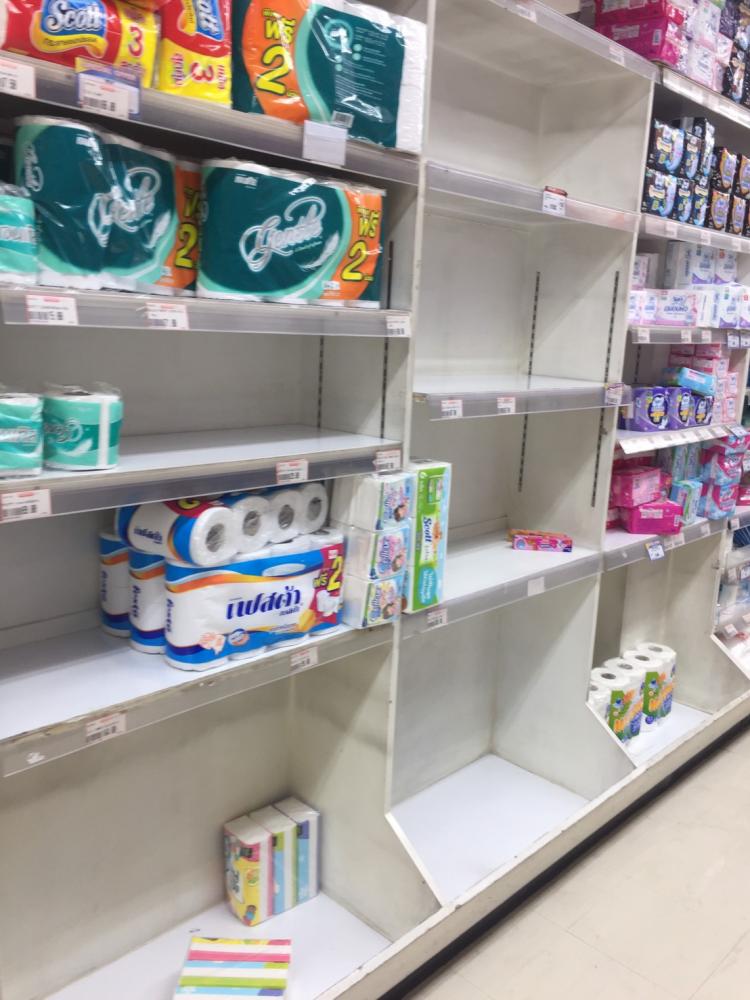This indoor photograph appears to capture a portion of a store's wall, showcasing various shelves and cubbies stocked with items for sale. The visible shelving is divided into three main sections. The first section on the left side of the image features five shelves, some of which are quite full while others are nearly empty. Among the stocked items, bath tissue is notable, although the brand names are illegible due to the image's blur. The middle section also contains five shelves, though the top shelf is partially cut off from view. Here, most of the shelves are empty, except for a few products on the second shelf from the ground. The final section, towards the right side of the image, has five shelves as well, and unlike the other two sections, most of these shelves contain products. These products, encased in boxes and plastic wrap, have price tags beneath them, though again, the blurry image makes the text difficult to decipher. The items appear to include bath tissue and possibly some medical-related products, given their packaging, although the blur prevents clear identification.